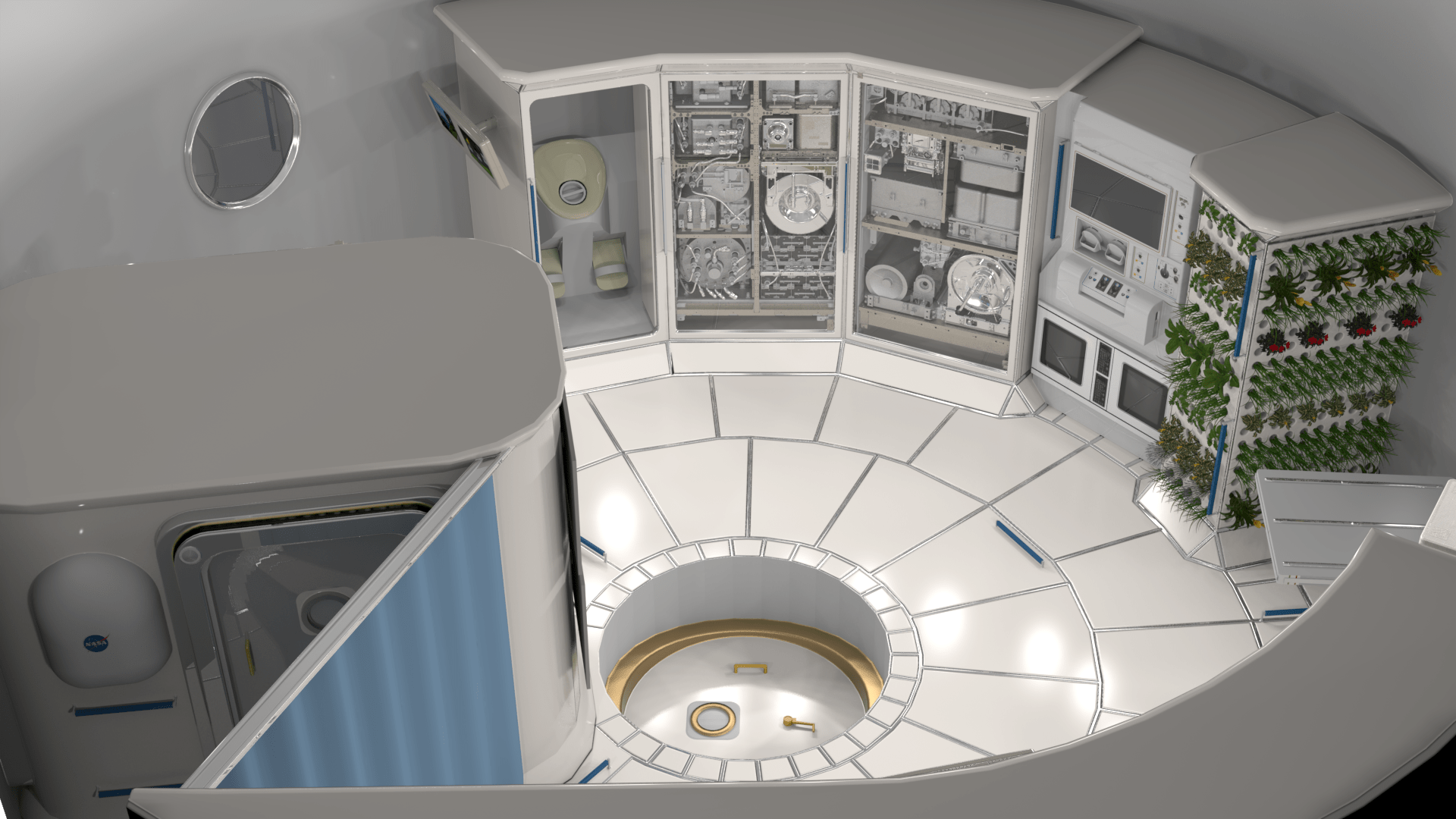The image depicts a room resembling an old-school control panel room or possibly a spaceship control center, taken from a high-angle perspective, about 20 feet above, looking down. The room has rounded beige walls and is well-lit. Dominating the center is an indented circular platform, about a foot deep, with white and gold accents, surrounded by pristine white tiles. This indentation gives the impression of an advanced piece of equipment, possibly a cylindrical structure. 

Encircling the room, primarily towards the back, are various control boards, switches, wires, and small computer screens, all hinting at high-tech usage - possibly scientific, medical, or electronic. To the left back corner is a round mirror above an area that might be another room or a control cubicle, adding to the futuristic atmosphere. Adjacent to it appears to be a sectioned-off area with a blue curtain and a silver door, resembling an elevator but likely serving a specialized purpose.

On the far right side of the image, part of a table with metal accents is visible, suggesting a workspace. Cabinets nearby hold what seem like mechanical parts and bottles, which might be substances or tools for experiments. Overall, the space exudes a clean, organized, and high-tech ambiance, indicative of a control or laboratory setting.